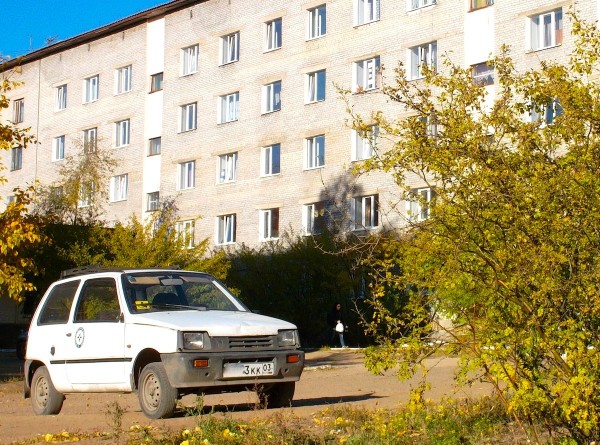The image captures a small white two-door hatchback parked on a dirt surface or possibly concrete. The vehicle is facing forward, showcasing its headlights and small yellow-orange lights, with a visible European license plate reading "3 KK 03." Its tires appear worn or dirty. A yellow sticker is noticeable on the right side of the front dashboard. To the right of the car is a close-up of a yellow and brown bush.

In the upper portion of the photograph, a large five-story cream or off-white brick building dominates the background. The structure features four vertical columns of rectangular windows, arranged in sections of six, with at least twelve visible windows. Surrounding the building are various plants, including trees and bushes, partially obscuring the lower part of the structure. 

A person is positioned near the bottom center of the photo, holding what appears to be a white bag. In the very top left corner, a small sliver of blue sky is visible, adding a touch of contrast to the scene.